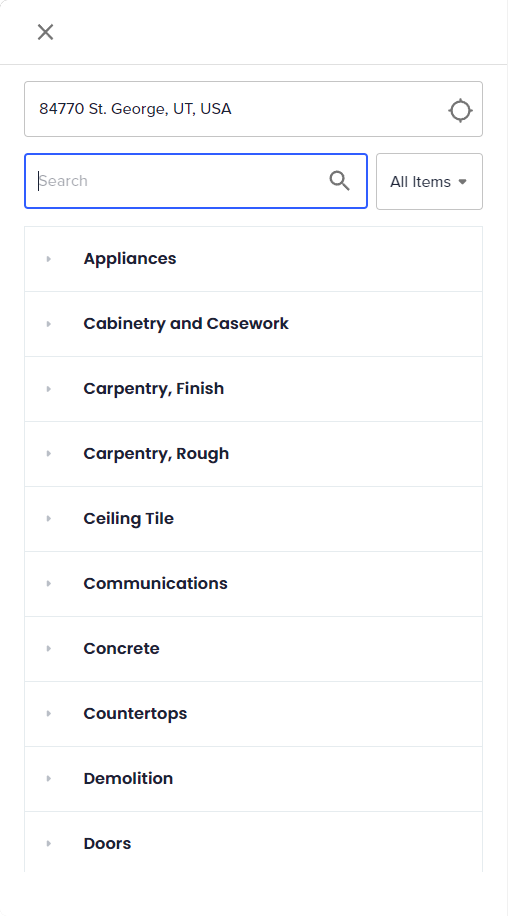The image is a screenshot taken from a cell phone, displaying a user interface with a clean, white background. At the top of the screen is a green "X" cross icon, likely representing a clothing category. Directly below this is a text box containing an address: "Annette, 84770 St. George, USA," written in black ink on a white background.

Further down, there's a search bar outlined in blue, accompanied by another bar labeled "All Items" with a dropdown arrow beside it, suggesting options for filtering content. 

Below these elements, there is a series of clickable options, each associated with different categories. These categories include "Appliances," "Cabinetry and Case Work," "Carpentry," "Fishing," "Roof," "Ceiling Tile," "Communications," "Concrete," "Countertops," "Demolitions," and "Doors." Each category name is preceded by grey bullet points and is written in bold black ink, denoting them as interactive links.